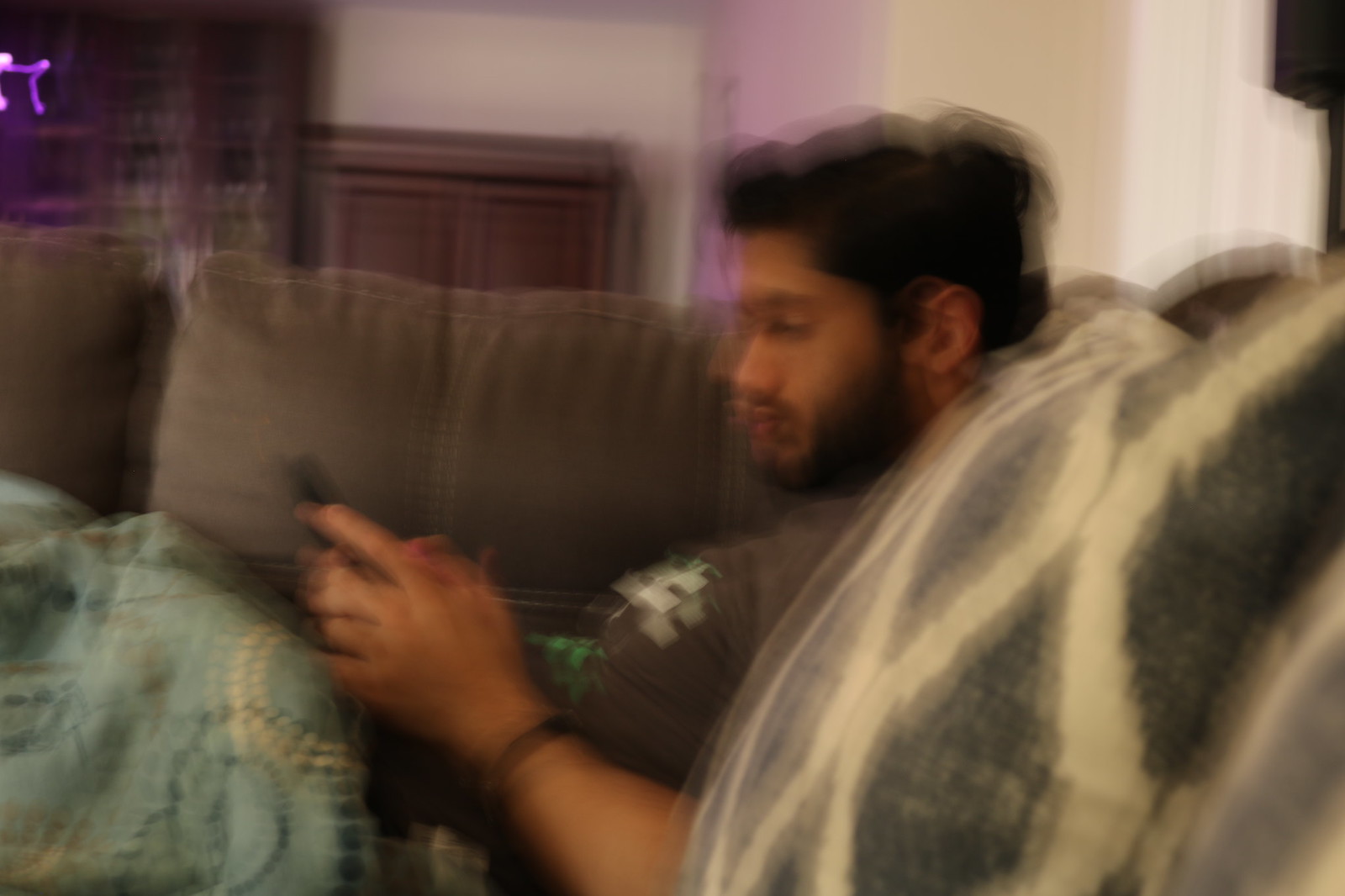The image captures a blurry scene of a man lounging on a gray couch, viewed from the side. The man, who has short black hair and a thick black beard, is looking down at a black cell phone, which he holds with both hands propped on his stomach. He's wearing a gray t-shirt that features some white lettering or patterns, which are hard to discern due to the blurriness. The shirt closely matches the tone of the couch. Wrapped around the man is a blanket that appears to be light blue with white and dark black stripes, possibly forming a floral pattern, though it's unclear. Additionally, he has a black bracelet or watch on his wrist.

Behind him, a white wall serves as the backdrop, contrasted by an entertainment stand and a smaller, flanking stand, both dark brown. An LED light on the main stand emits a purple glow, which also appears in the top left corner, possibly from a neon sign, sheer curtain, or another source of illumination. Adding to the scene is a dark gray pillow with white stripes situated to the man's right on the couch.